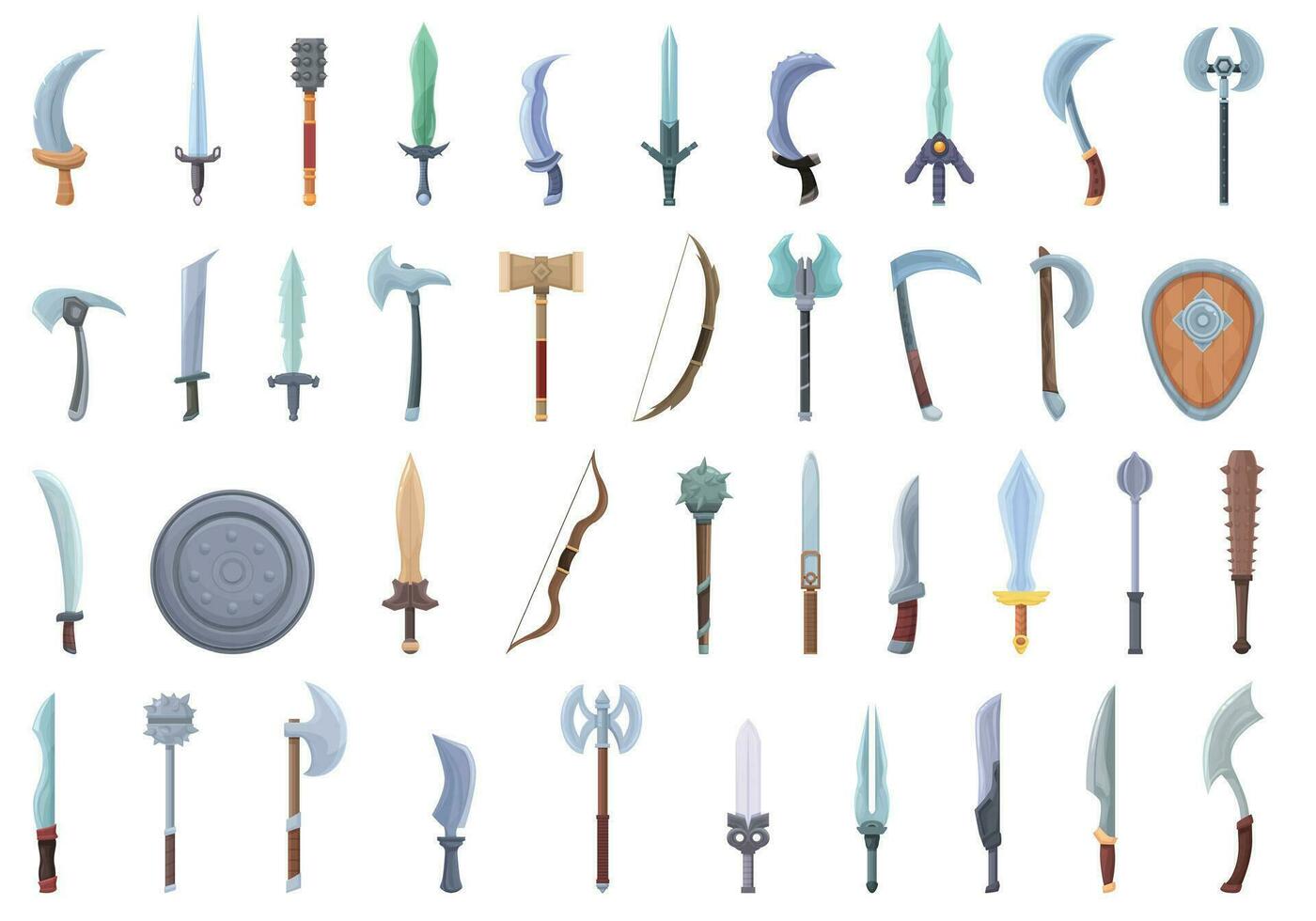This is a detailed, colorful illustration showcasing an assortment of approximately 50 medieval and fantasy weapons, likely designed for a video game. Displayed against a white background in a clean, simplified style, the weapons are evenly spaced and organized into four rows with each row containing around 12 items. The top row primarily features various daggers and swords, including some with curved and straight blades, as well as a distinctively studded mace. The second row displays an array of scythes and axes, along with a jagged sword, a broad blade sword, a crossbow, and a wooden shield trimmed with metal. The third row contains more unique items, such as a pirate-like cutlass, a round Viking shield, another bow, a cat o' nine tails type mace, and a spiked bat reminiscent of Negan's weapon from The Walking Dead. The bottom row continues the theme with additional battle axes and comparable medieval weaponry. The blades predominantly feature silver or light blue hues mixed with gray, while the maces, hammers, and clubs are multicolored. One shield is entirely silver, while another combines silver trim around a wooden base with a floral emblem at its center.